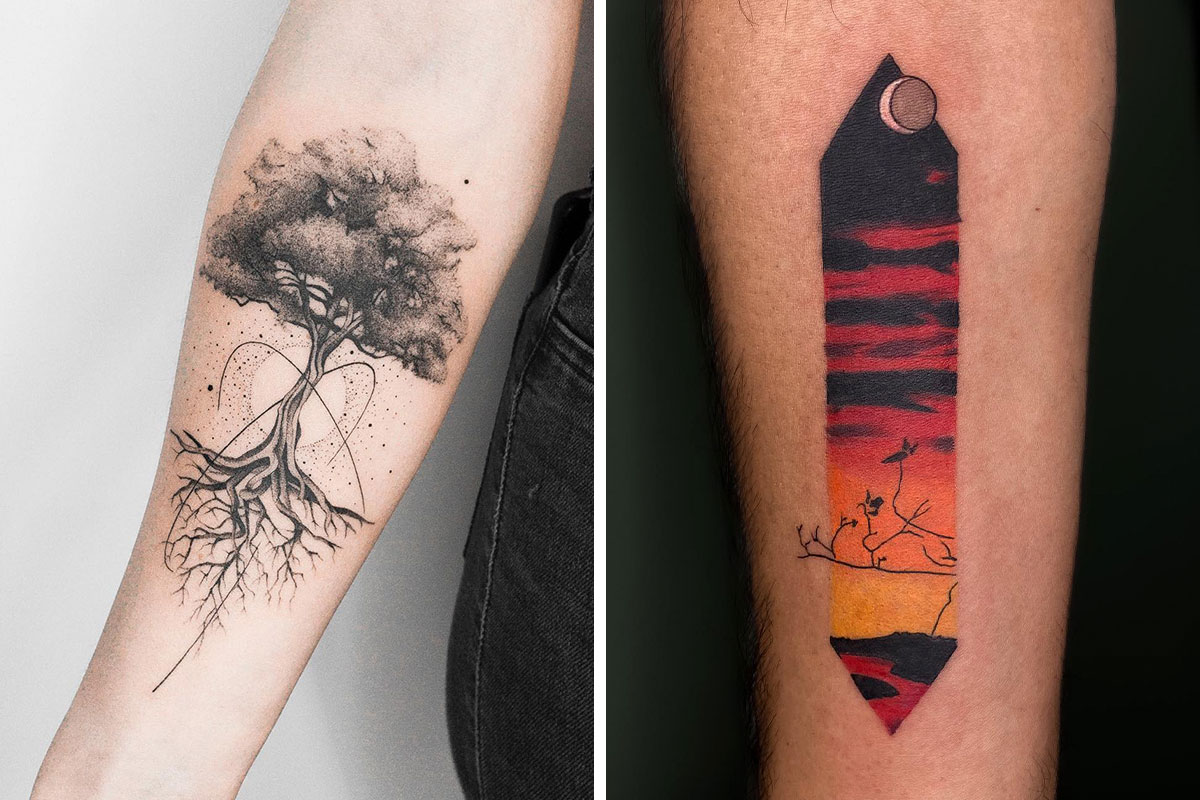The image showcases two tattoos on forearms, positioned side by side against a white background. The left arm, likely belonging to a female, features a detailed black-and-white tattoo depicting a tree with visible roots and a canopy treetop. Behind the tree is a sun, intersected by two diagonal lines. The right arm, of slightly darker skin tone, displays a vibrant, colorful tattoo shaped like a tie with pointed ends. The design transitions from a black and red sky to an orange horizon, with a red river flowing through a scenic landscape that includes tree branches and birds.